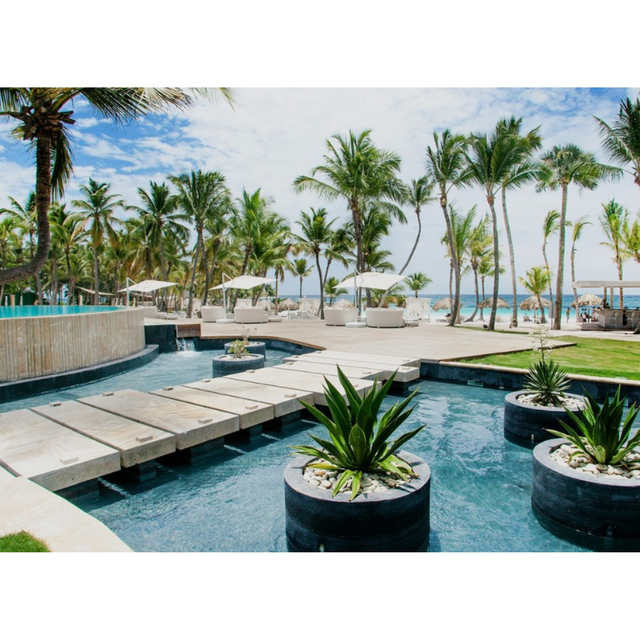The image showcases a luxurious beachside resort, predominantly featuring the resort grounds with only a partial glimpse of the beach in the background to the back right. A wooden plank bridge extends from just above the bottom left corner toward the center, flanked by shallow blue water on either side. Floating in the water are dark gray, cylindrical pots filled with white stones; these pots support green spiked plants and, to the left, some brown plants. To the left of the bridge, there is an elevated platform enclosed by a light blue glass fence, and behind it, a cluster of tall palm trees with gray trunks and green fronds. On the right side of the bridge, white lounge chairs are shaded by umbrellas, adjacent to a small grass lawn. The sky above is mostly covered in white clouds, with patches of blue visible on the top corners. Overall, the photograph captures a serene and elegant outdoor scene during the daytime, highlighting the opulent amenities and natural elements of the resort.